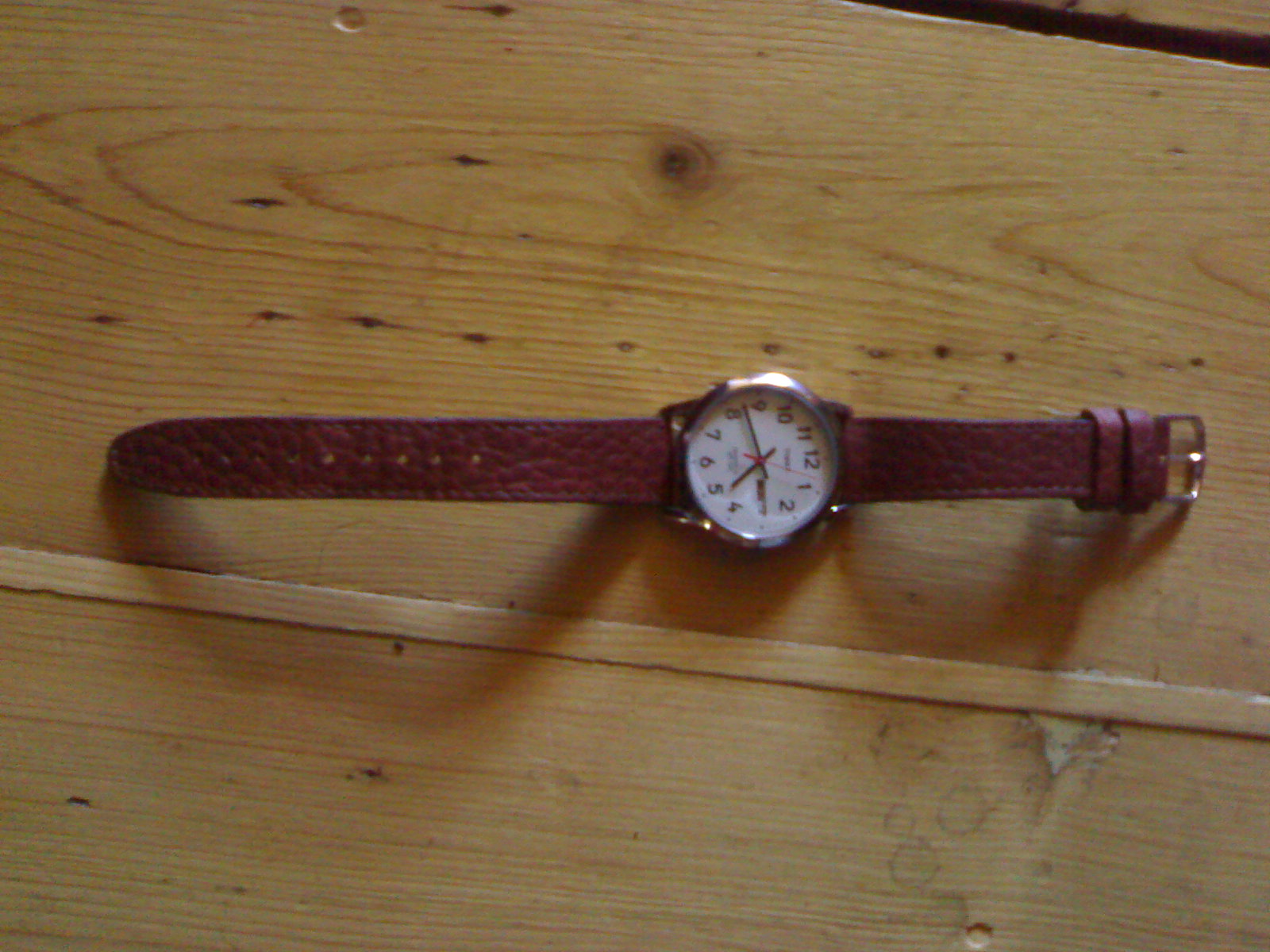This rectangular, horizontally elongated image features a wooden piece of furniture with a natural brown stain. Positioned centrally on the furniture is an elegant lady's watch. The watch has a thin, textured brown leather band adorned with gold hardware. Its round white face displays the time at 4:45 with the numerals 12 positioned at the top and 6 at the bottom. The red second hand is situated between the 12 and 1. A shadow of the watch is cast upon the wooden surface, adding depth to the composition.